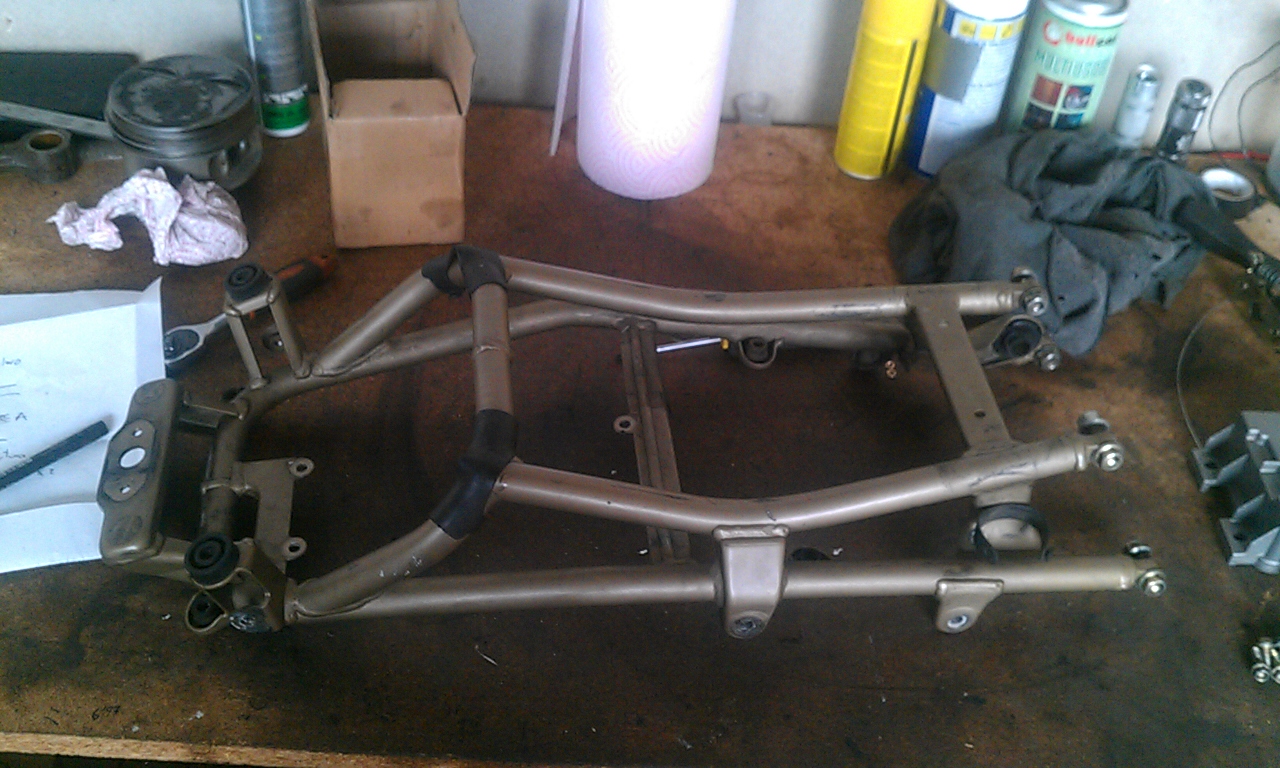The photo, taken indoors, features a cluttered brown workbench against a white wall. Dominating the workbench is a metal contraption resembling a small walker, though it lacks an opening at the back, hinting it might serve a different purpose. The device appears partially disassembled or broken, with some areas held together by duct tape. Scattered around the workbench are various items: a white piece of paper with a pen on it, a used paper towel, a fresh roll of paper towels, black duct tape, a small flashlight, a t-shirt or cloth, and several spray canisters in green, yellow, and white. A cardboard box, seemingly empty, also lies nearby, adding to the disarray of the workspace.